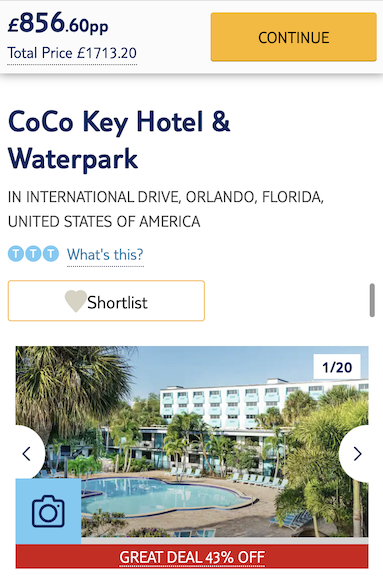Screenshot of the booking page for Cocoa Key Hotel and Waterpark located on International Drive, Orlando, Florida, United States of America. The total price for the entire stay is displayed as £1,713.20, with an individual rate of £856.60. In the top right corner, a yellow 'Continue' button is prominently positioned. The hotel's name is highlighted in large navy blue font, and detailed information about its location follows in small black font. Three 'T's inside blue circles are accompanied by a clickable 'What's This?' link. Below, an option to 'Shortlist' the hotel, with a heart icon next to it, is encased in a thin orange border. The main image, labeled as image 1 of 20, showcases the hotel’s pool set in the center with the building and surrounding palm trees. A camera icon is located at the bottom right of the image. A red bar at the bottom of the screen with white font announces a "Great Deal: 43% Off." The background is predominantly white with most of the text in black.